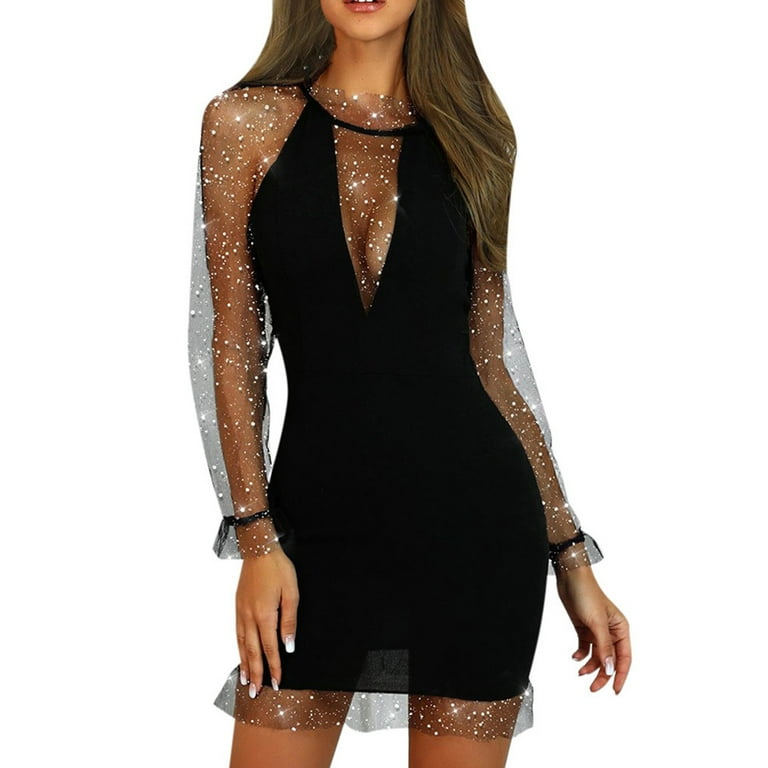The image showcases a model against a solid white background, highlighting her attire from just below her lips to her thighs. She is wearing a striking black cocktail dress with a deep V-shaped neckline, elegantly accentuating her curves. The dress features two thin shoulder straps and hugs her figure tightly. The fabric includes chiffon-like sheer sections on the long sleeves and the lower part of the skirt, which is adorned with silver glitter, creating a sparkly effect. Her straight, long brown hair cascades over one shoulder, complementing the overall glamorous look. The dress's see-through elements on the sleeves and chest area enhance its sophisticated yet alluring appeal.